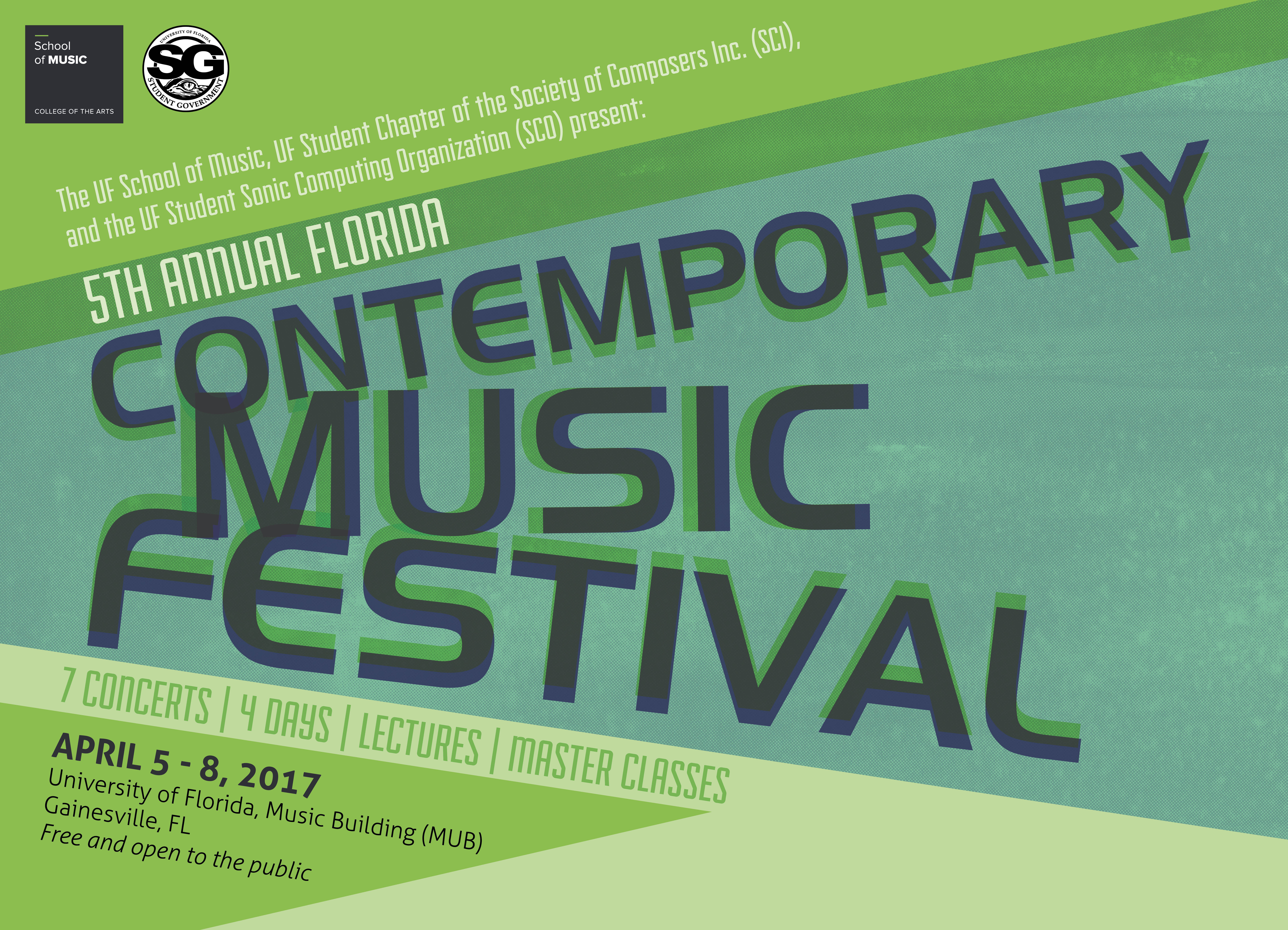**Detailed Caption:**

This image is a display advertisement for the "Fifth Annual Florida Contemporary Music Festival." The ad is designed with a visually striking layout, featuring a prominent headline arranged in a unique triangular format. The word "Contemporary" is written at the top in bold, blue capital letters, outlined in green, with a slant towards the upper right-hand corner. Beneath it, the word "Music" appears almost horizontally, providing a contrast to the slanted elements. The word "Festival" is positioned at the bottom, slanting towards the bottom right-hand corner.

At the very top, within a green border, the ad features a white text that reads, "Fifth Annual Florida," indicating the event's edition and location. The advertisement's background is a light green, enhancing readability and adding to the overall aesthetic. 

In the bottom left-hand corner, detailed event information is provided, including the dates "April 5th through 8th, 2017." The venue is clearly mentioned as the "University of Florida Music Building (MUB), Gainesville, Florida." The ad also emphasizes that the event is "Free and Open to the Public."

This eye-catching design and detailed informational layout effectively promote the upcoming music festival, ensuring that all pertinent details are easily accessible to viewers.